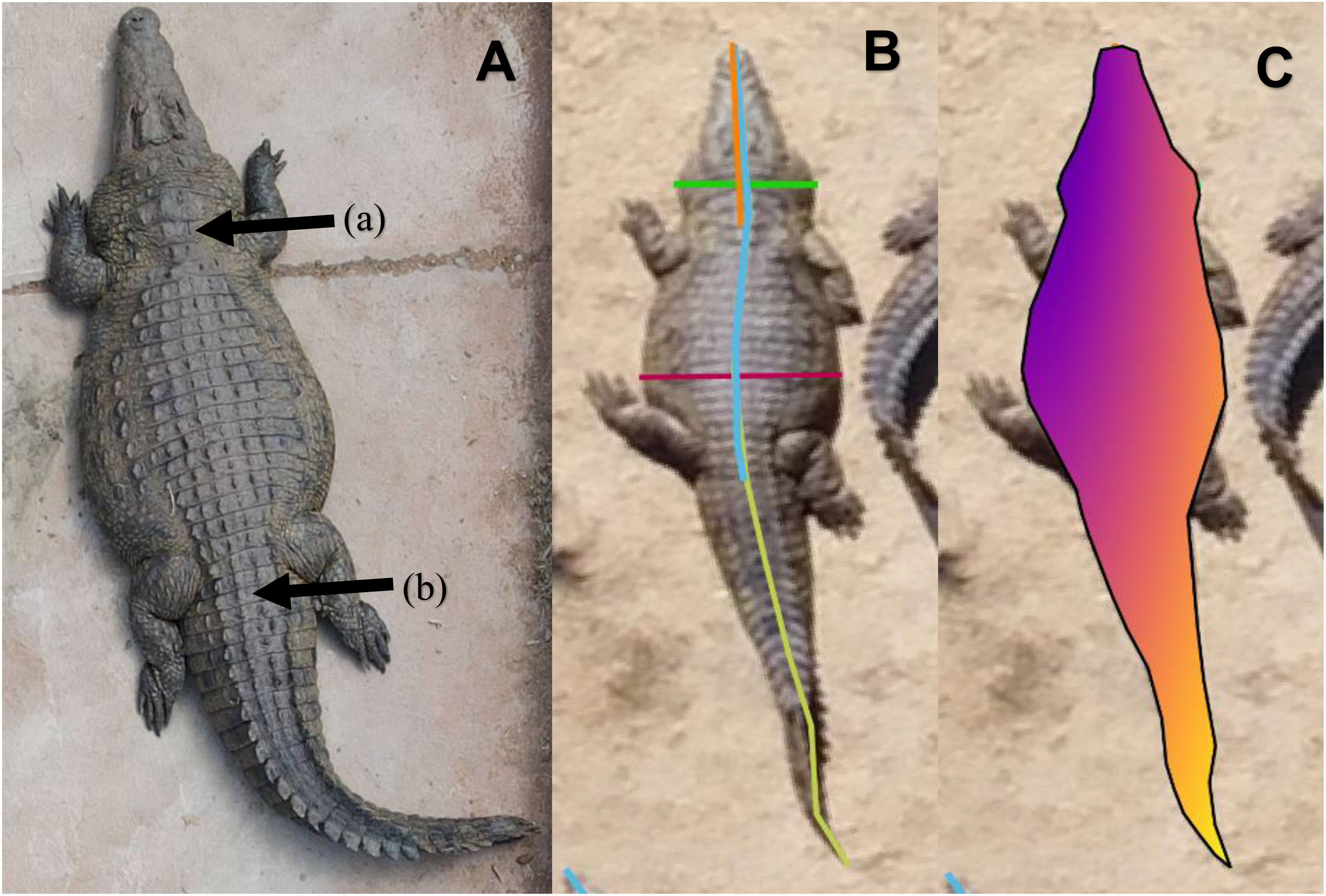This is a detailed scientific diagram in color featuring three horizontally divided sections labeled A, B, and C, each showing an aerial view of an olive green alligator on a light brown, flat surface. Section A, on the left, depicts the alligator viewed from above with two black arrows: one labeled "A" pointing to the back of its neck and another labeled "B" pointing to the base of its tail. The alligator has short, stubby legs, and its tail curves slightly to the right.

In the middle, Section B displays the same alligator with distinct color lines drawn on its body: a blue line runs vertically from the tip of its snout to the base of its tail, which is marked by a yellow continuation. Additionally, a green line crosses horizontally at the neck, while a red line intersects the abdomen.

Section C, positioned to the right, presents the same alligator image overlaid with a color gradient outline resembling a heat map. This outline transitions from purple at the head through orange in the midsection, finally fading into yellow down the length of the tail. The entire diagram is set against a black background, enhancing the visibility of the annotations and lines.